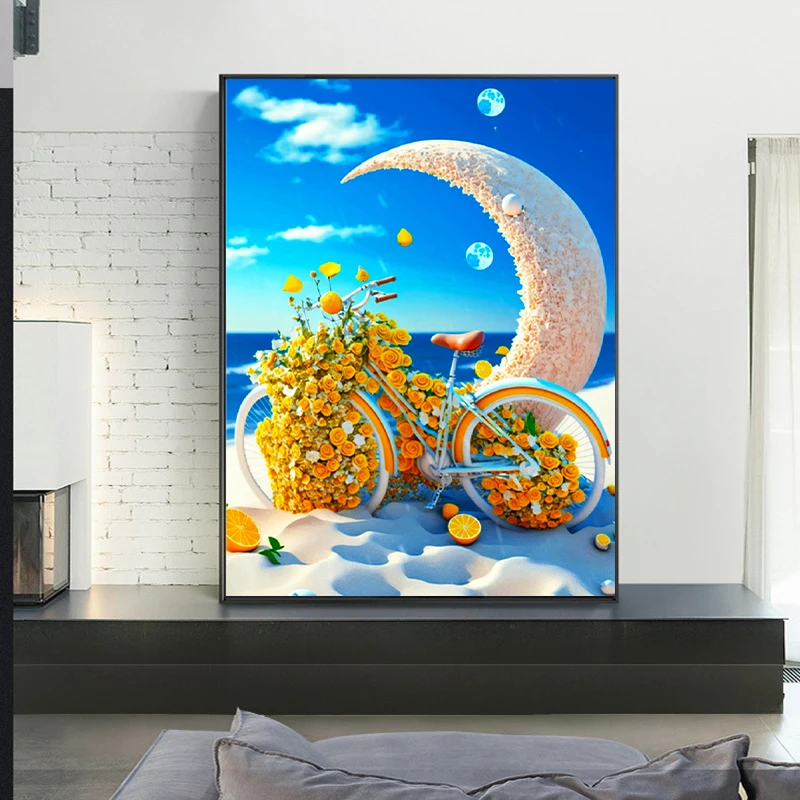The image captures a painting prominently displayed in a modern living room with abundant natural light filtering through sheer white curtains. The painting, large and vibrant, rests atop a long, gray bench-like structure against a white brick wall, resembling a fireplace mantle without the actual fireplace. The room has a sophisticated aesthetic, complete with a hardwood floor and a grey couch in the foreground.

The artwork itself depicts a surreal scene featuring a vintage blue bicycle with a red seat, akin to a mid-20th-century beach cruiser. The bicycle is adorned with a profusion of orange flowers, cascading from the front wheel through to the handlebars and back wheel, blending seamlessly with the composition. Scattered around the white sandy beach in the foreground are halved oranges, adding a whimsical touch. Behind the bicycle, a large crescent moon hovers close to the horizon, its texture reminiscent of an orange peel's white membrane. Two additional moons — one near the horizon and another high up in the sky — enhance the dreamlike atmosphere of the scene. The sky is a vivid blue with occasional wisps of white clouds, and a serene blue ocean stretches out beyond the bicycle.

To the left of the painting, partially cut off, is a white box with glass, resembling an aquarium case, though its function is unclear. Overall, the painting's colorful and fantastical elements vividly pop against the neutral tones of the modern living room, making it the focal point of the space.